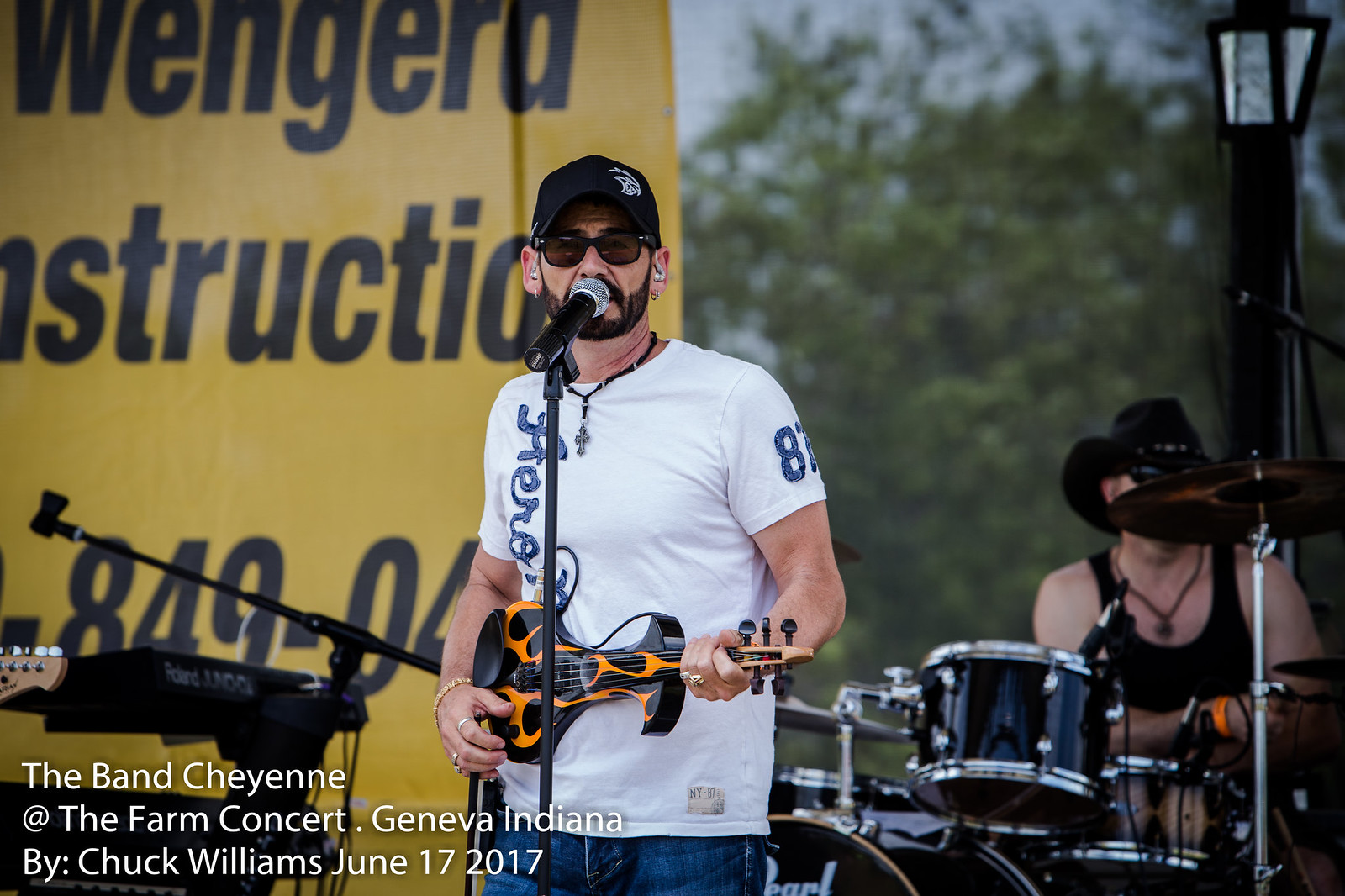In this detailed image, we see an outdoor music concert taking place in the middle of the day. Central in the image is a man singing into a microphone, strumming a black and orange electric guitar. He is wearing a black hat, sunglasses, a white t-shirt with "83" printed on the left bicep, and blue jeans. Directly behind him is a yellow banner with the text "Wingard Instruction" in large black letters. To his right, we see a full drum set being played by a drummer dressed in a black tank top, black cowboy hat, and sunglasses. Off to the right, there's a lantern in front of a tree, and at the top right, there are glimpses of the blue sky and more trees. Additionally, there's a sign on the left mentioning "WENGERA" and possibly more text obscured, linked to construction, reading "849-04." Also on stage are a second guitar and a keyboard. The bottom left of the image contains white text that reads, "The Band Cheyenne, The Farm Concert, Geneva, Indiana, by Chuck Williams, June 17, 2017." The various colors in the image include black, yellow, white, brown, silver, orange, blue, gray, and green. Overall, the setting is lively and vibrant, capturing the essence of a live performance.